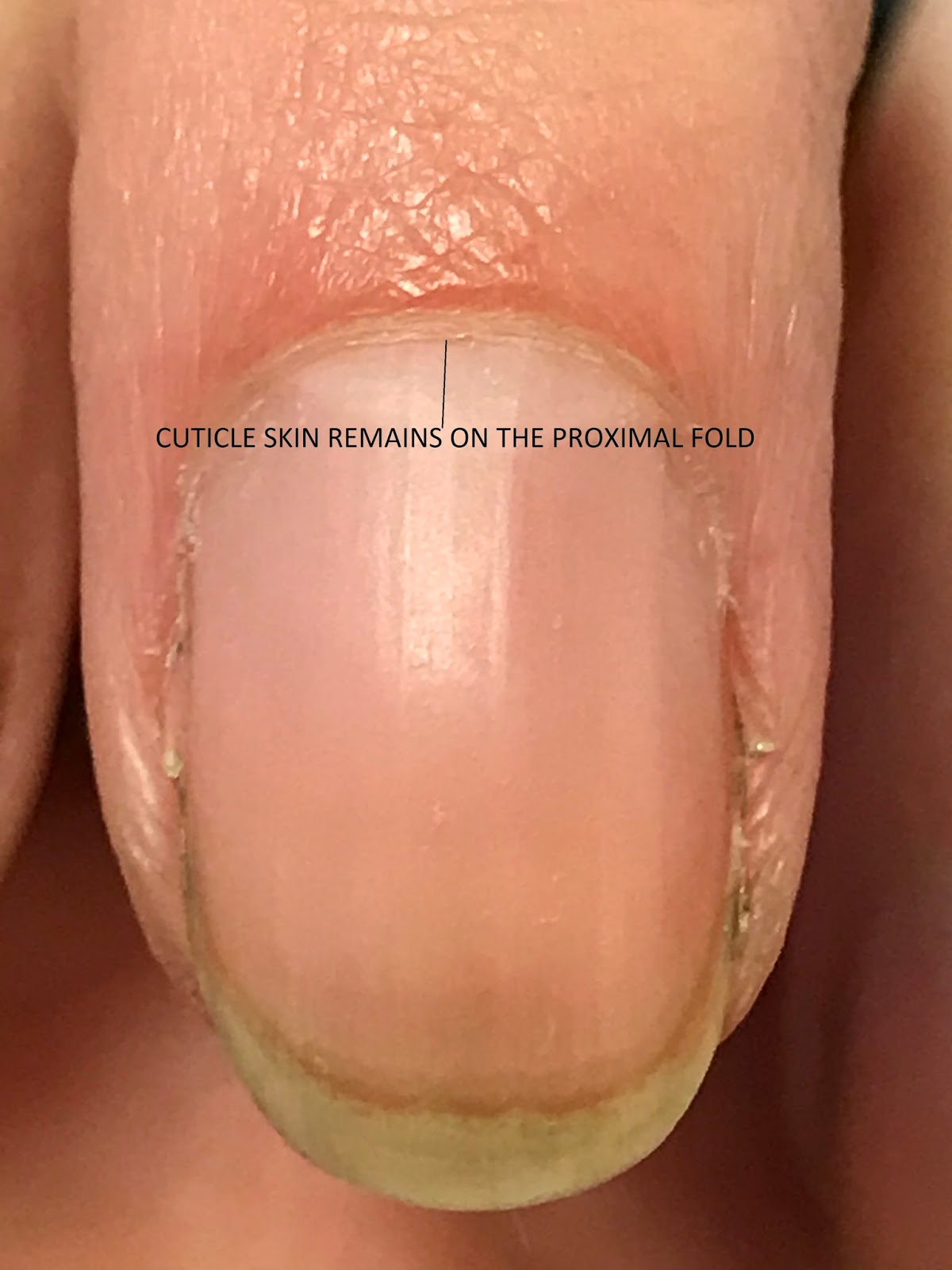This high-resolution close-up image features a Caucasian finger with a yellow-brown fingernail, indicating it hasn't been cleaned recently. The nail appears slightly reflective with minimal striations and shows some white at the tip. The surrounding skin exhibits dry areas, creases, and a pronounced, whiter cuticle. There is visible dirt under the nail. Black capital letters with a thin line pointing to the cuticle read, "cuticle skin remains on the proximal fold," suggesting the image serves an educational purpose. The background fades to an out-of-focus, darker hue, and parts of adjacent fingers are visible on either side of the image.